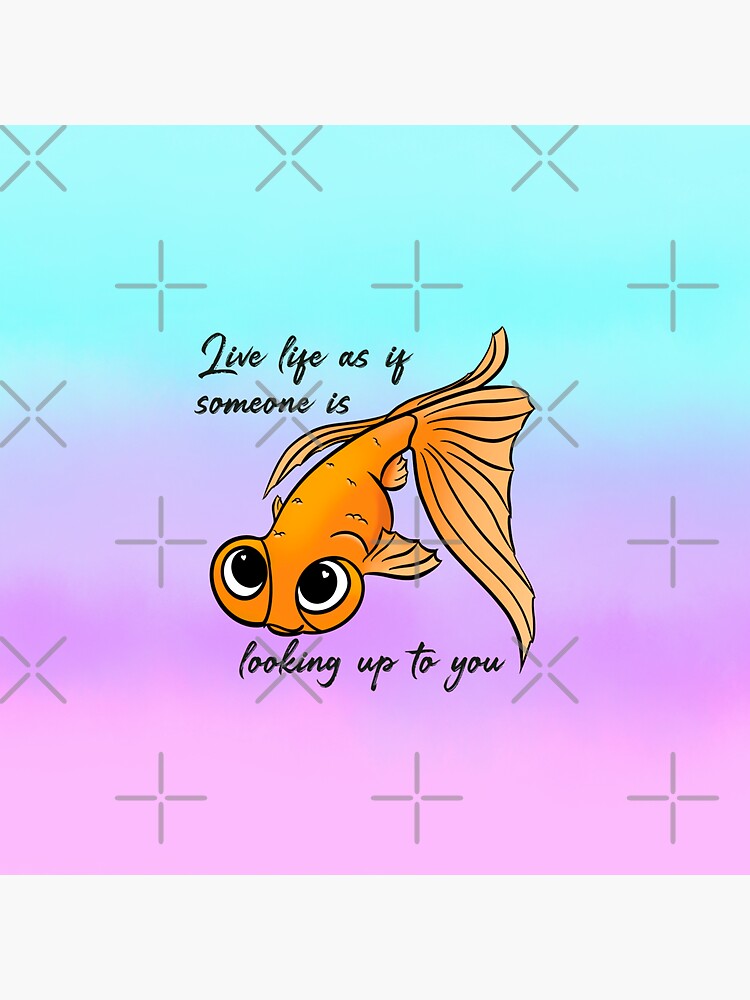The image is a square clipart with a pastel gradient background, transitioning from aquamarine at the top to lavender in the middle, and finally to pink at the bottom. Overlaid on this softly blended background are gray X's and crosses, possibly indicating a transparent watermark. 

At the center is a cartoonish, pen-and-ink drawing of a goggle-eyed goldfish, its large, bulging eyes gazing directly at the viewer. The goldfish is colored in orange, with its fan-shaped tail trailing off to the right. Above and below the goldfish, in black script, is the motivational phrase: "Live life as if someone is looking up to you." The artwork does not bear any artist's signature or mark.